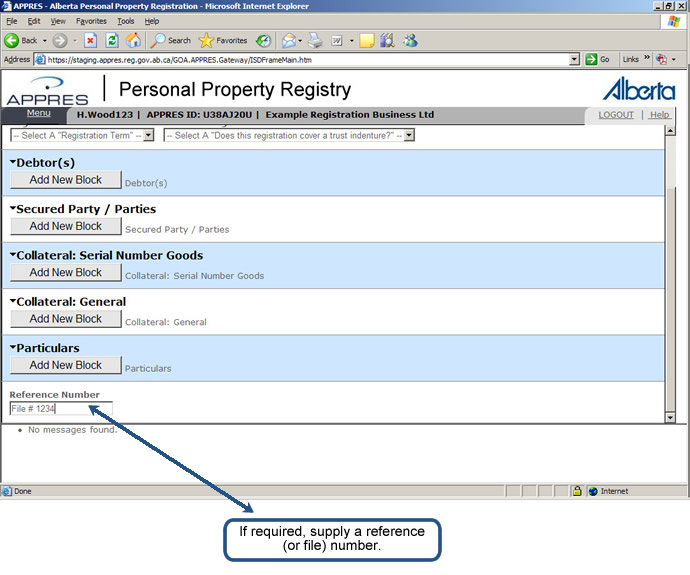Screenshot of an older version of Internet Explorer displaying the Alberta Personal Property Registration website. The interface shows a government registry page on a staging environment at staging.appres.reg.gov.ca, indicating it's a Canadian site. The page allows users to input information about debtors, secured parties, and collateral particulars, which are likely related to the processes of personal property registration. The design scheme features a blue and white color palette with dated UI elements typical of the 1990s web design, reflecting the legacy look of the browser and the software.